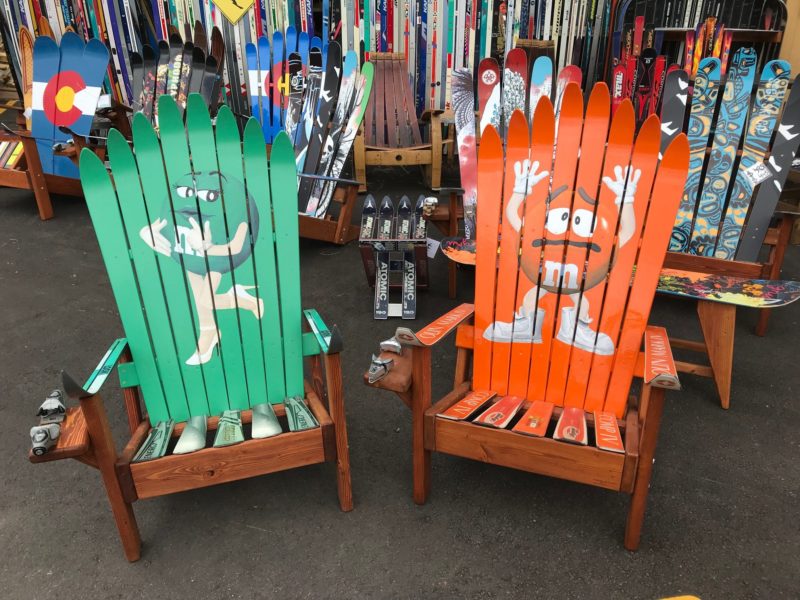This image depicts an outdoor display of several Adirondack-style chairs, likely from a surf supply or outdoor furniture shop. The chairs are arranged on a paved surface, with the focus on two prominent front-row chairs featuring painted M&M characters. The chair on the left showcases the green M&M, characterized as a feminine figure with white high heels, white gloves, and long white eyelashes. The backrest of this chair is painted green. To the right, the chair displays the orange M&M, noted for its scared expression, white sneakers, and white gloves, set against an orange background. The chairs are made from repurposed snow skis, evident from the ski shapes used in both the backrests and seat bases, with some having brand markings like "Atomic." Behind these two main chairs are others with various designs including a blue and yellow tribal pattern, a mountain scene, and a Colorado State flag depicted on a chair with a blue back, white stripe, and red "C" encircled with yellow. Another partially visible black chair hints at a costumed figure, adding to the eclectic, artistic display.